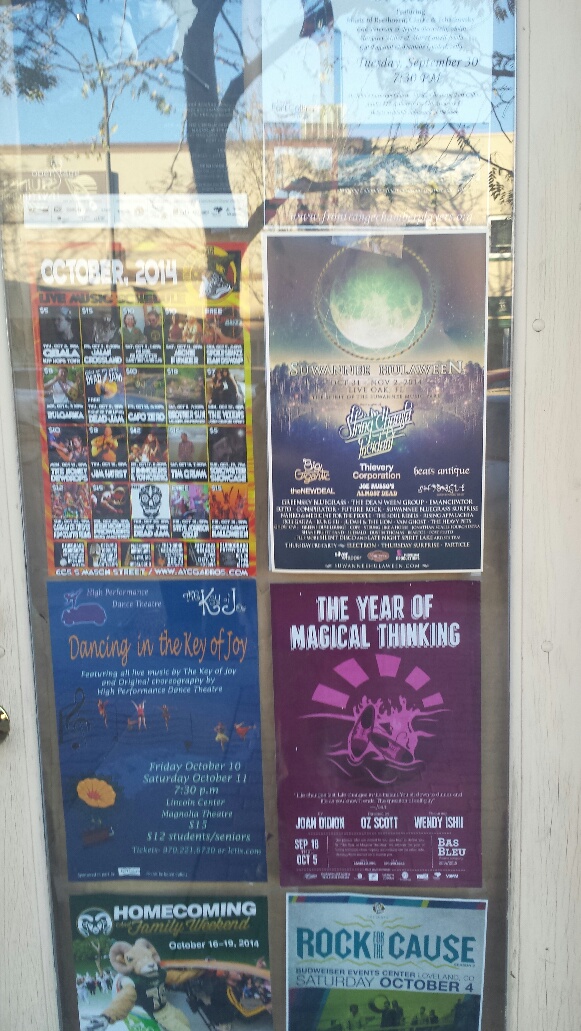The image shows a storefront window filled with an array of posters, partially obscured by reflections. The door to the shop is visible on the left side of the frame, crafted from grayish-white wood with a rounded top that's cut off by the image's edge. It features a glass panel adorned with a variety of colorful flyers and posters. These pieces of advertisement display a blend of themes, including events and performances from October 2014.

Central among the posters is an announcement for "Dancing in the Key of Joy," presented by the High Performance Dance Theater, detailing jive music and original choreography with performance dates listed as Friday, October 10th, and Saturday, October 11th, at 7:30 PM at Lincoln Center's Magnolia Theater. Nearby, another prominent flyer proclaims "The Year of Magical Thinking" against a purple background with an ambiguous musical instrument illustration.

The scene also includes posters for additional events such as "Rock for the Cause" at the Budweiser Events Center in Loveland, Colorado, on Saturday, October 4th. Further details mention a "Homecoming Family Theater" and a glimpse of a poster for a "Hulaween" event on the right side. The entire setup suggests an outdoor setting in the middle of the day, with vibrant reflections cast across the windowblasting an array of colors including purple, pink, white, yellow, green, and blue.